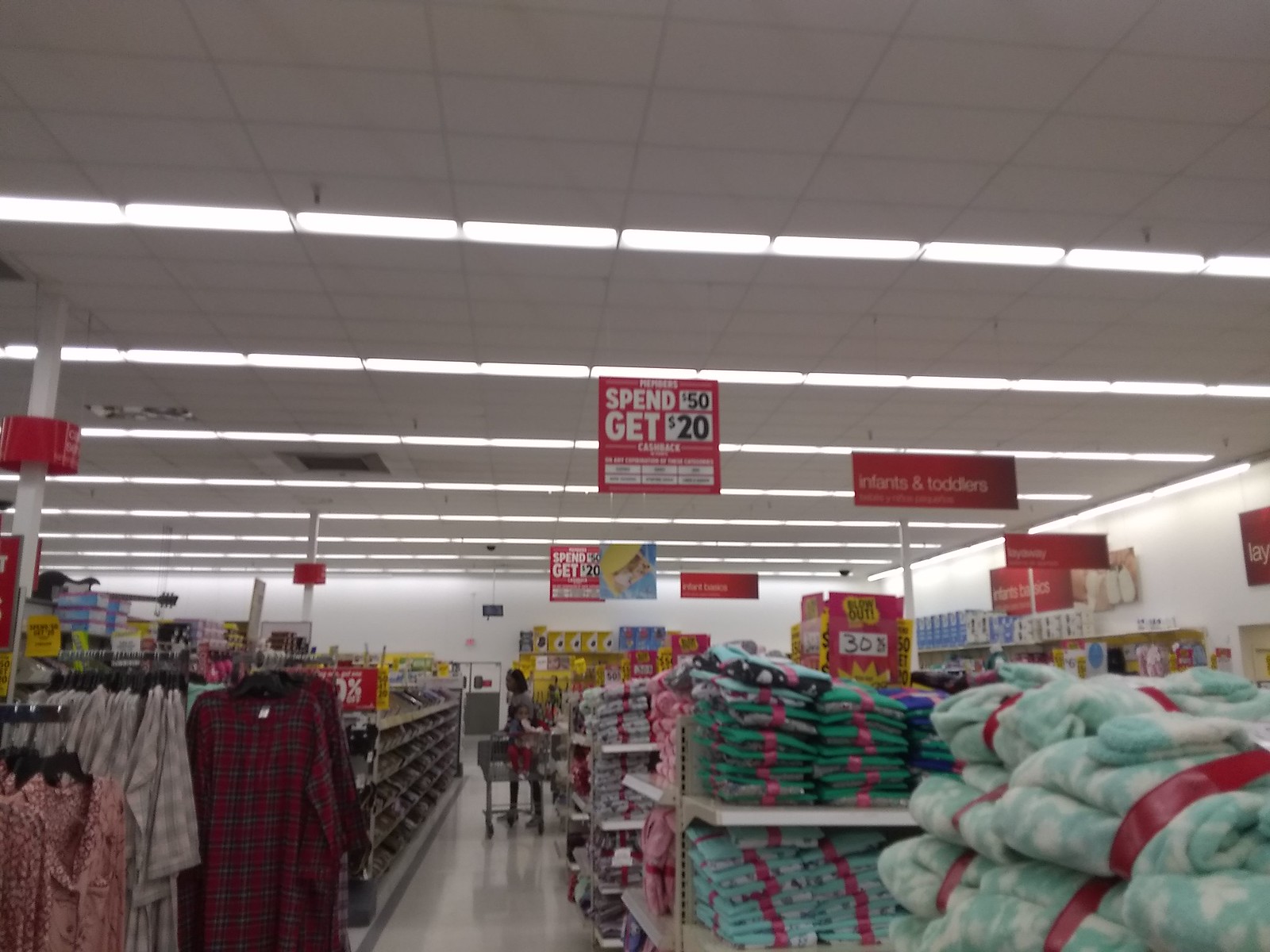This photograph captures the interior of a department store, showcasing a bright, spacious shopping environment. The store features pristine white walls, a drop ceiling with light gray square dividers, and commercial-style fluorescent lights arranged in horizontal rows, bathing the space in steady illumination. Prominent signage hangs from the ceiling, including a red promotional sign in the center displaying "Spend $50, Get $20 Cash Back" in bold white letters. Another sign indicates the "Infants and Toddlers" section. 

In the foreground, modular shelving units are filled with various fleece blankets in colors such as green, white, teal, and pink. To the left, racks are neatly lined with women's robes and nightgowns in red and blue plaid. Further into the store, racks display a collection of shirts and folded comforters or blankets.

A solitary shopper, wearing pink shorts, navigates the aisles with a shopping cart, pausing to examine a rack of shoes. The overall atmosphere is orderly and inviting, typical of a well-organized retail space.